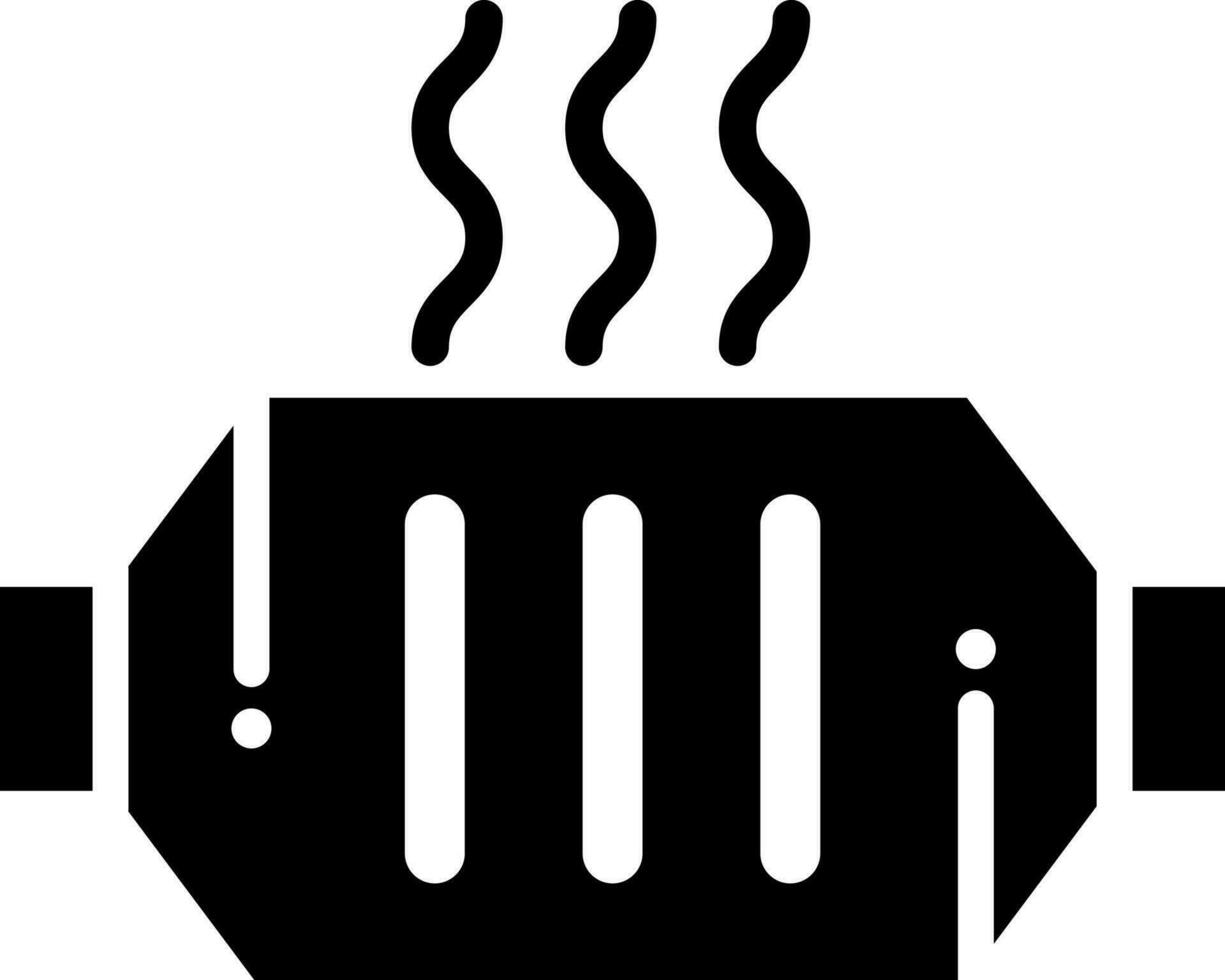This image portrays a minimalist, black-on-white illustration reminiscent of a Jeep grille. At the top of the image, three evenly spaced, black squiggly lines suggestive of smoke are symmetrically positioned. Below, the design features a frontal view of what appears to be a stylized Jeep grille. Two substantial, vertical black bars on either side of the image likely represent fenders or tires. Centrally positioned between the bars, the grille consists of three prominently exaggerated, elongated ovals with rounded edges, further enhancing the Jeep-like appearance. The entire composition stands out starkly against a transparent white background, emphasizing its simple yet evocative design.